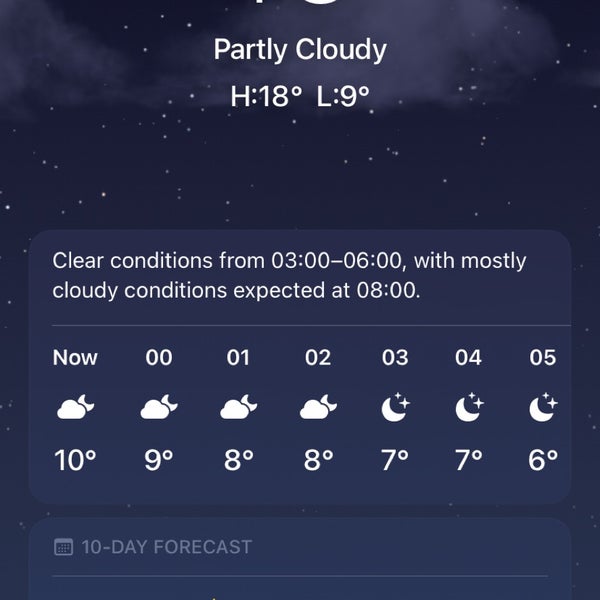This is a screenshot of a weather app displaying the current nighttime conditions. The background features a night sky with stars and clouds, indicating it is partly cloudy. The temperature shows a high of 18 degrees and a low of 19 degrees, though it is unclear whether this is in Celsius or Fahrenheit. Below, a detailed hourly forecast indicates clear conditions from 3 AM to 6 AM, transitioning to mostly cloudy conditions by 8 AM.

Icons illustrate the weather for each hour:
- At midnight (00:00), a cloud and moon icon with a temperature of 9 degrees.
- At 01:00, a similar cloud and moon icon appears with the temperature dropping to 8 degrees.
- The pattern continues at 02:00 with the same icon and an 8-degree reading.
- At 03:00, the icon switches to a moon and stars, showing 7 degrees.
- The moon and stars persist at 04:00 and 05:00, with temperatures of 7 degrees and 6 degrees respectively.

At the bottom of the screen, a partially visible "10-day forecast" text is cut off, leaving the extended forecast inaccessible in this view. This image provides a concise overview of the current and short-term nighttime weather conditions.